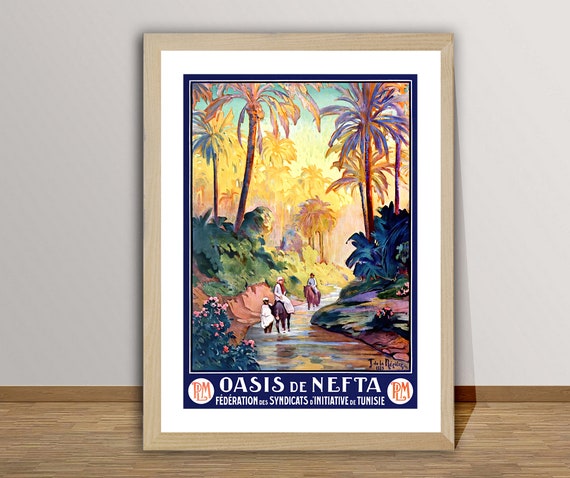This is an image of a framed watercolor painting, propped against an off-white wall with oak hardwood flooring and wood molding. The wooden frame of the painting is light brown, complemented by an inch-thick white border and a thinner dark blue border framing the artwork itself. At the bottom of the painting, white text reads "Oasis de Nefta, Federación Sindicats Iniciativa de Tunis." The scene within the painting depicts a lush, sunlit landscape with palm trees in the background and a river flowing through the center. Along the riverbanks, green bushes adorned with red flowers can be seen. Three individuals feature prominently in the foreground: two are on horseback, clad in white robes, with one wearing a red scarf. A third person, also in white, walks beside one of the dark-colored horses. The background is vibrant with various shades of green and brown, featuring plant life and a mix of landmasses that frame the river. Logos are positioned on each side of the descriptive text.